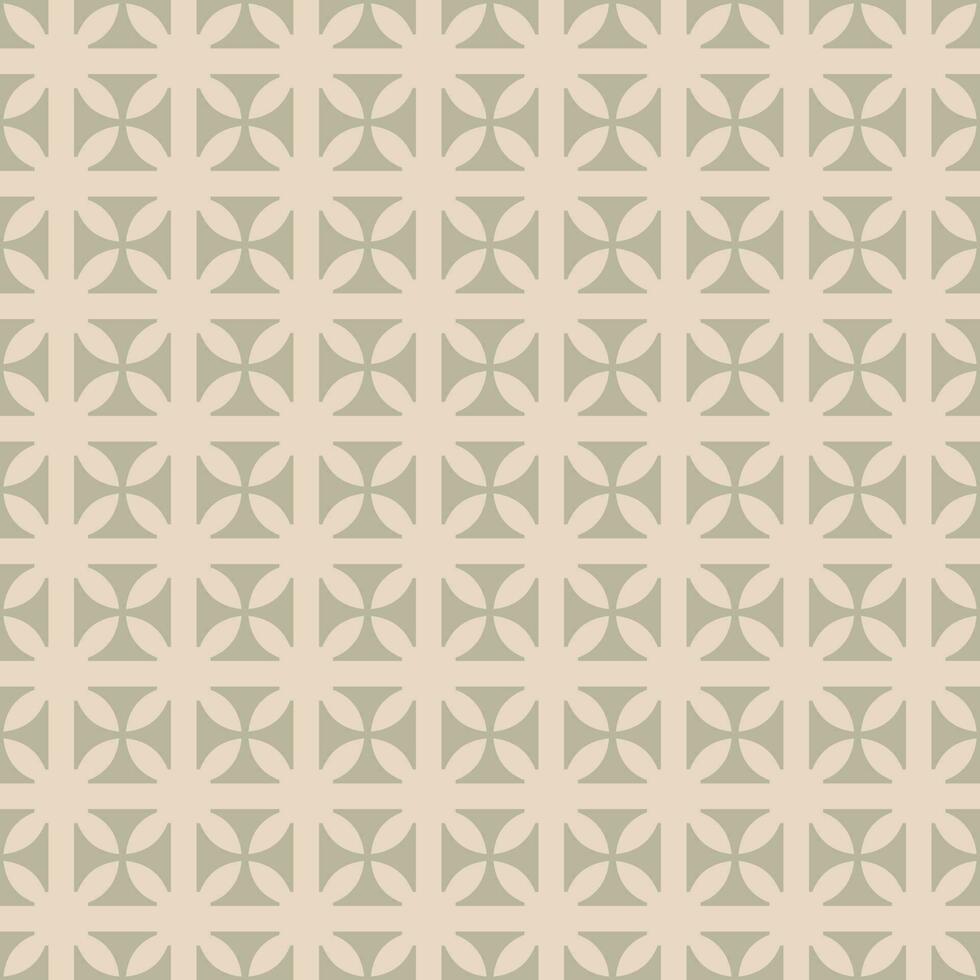The image presents a uniform and aesthetically pleasing repeating pattern set against a background that is described as a light, dusty sage color. The pattern itself is primarily a light cream tone. Depending on your focus, the design can transform visually. If you concentrate on the cream elements, you see a grid where each junction has a small protrusion creating a leaf-like shape. On the other hand, focusing on the sage areas reveals an intricate, medieval-style cross, reminiscent of a Templar cross. These crosses are narrow at their intersections and flare out towards the ends, forming a T shape. Additionally, the pattern can appear as plus signs with expanded edges tapering to meet at the center, or alternatively, the background can create the illusion of sprays of leaves or flowers with vertical and horizontal lines woven through them. This versatile design has a light, dusty sage background with intricate cream patterns that create a simple yet elegant overall effect.